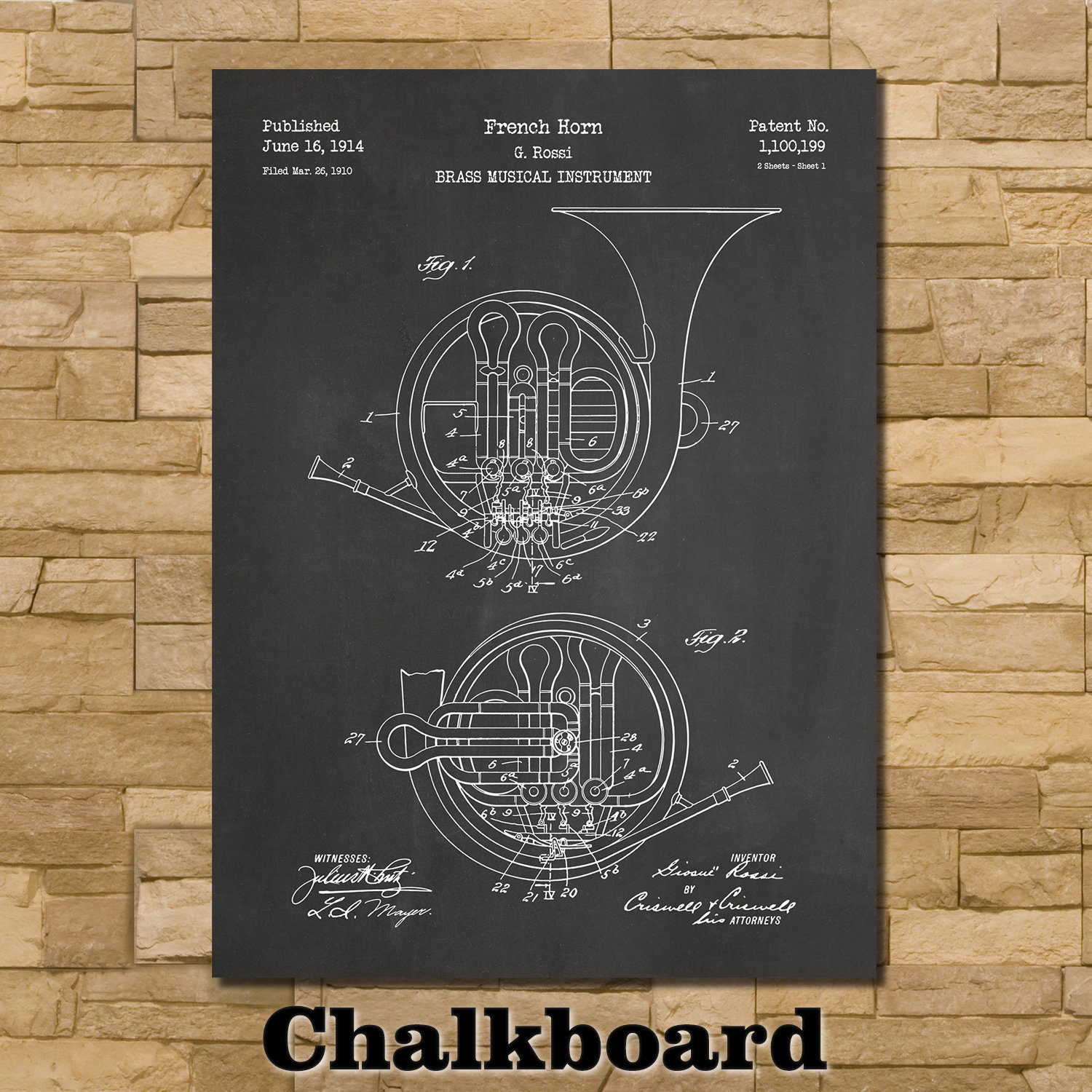This color photograph, presented in a square format, captures a detailed and historically significant placard mounted on a beige, stack stone wall. Central to the image is a vertical rectangular black placard with a chalkboard-like appearance. Dominating the placard are two intricately detailed white illustrations of a French horn, labeled as "Fig. 1" and "Fig. 2," showcasing various parts of the musical instrument. To aid in understanding, the illustrations are annotated with numbers pointing to specific sections, detailing areas such as the mouthpiece and finger placements, and these numbers range into the 30s.

At the top of the placard, text in white states, "French Horn G. Rossi Brass Musical Instrument," followed by the patent number 1,100,199. The left side reads "Published June 16, 1914," and also includes the filing date, "March 26, 1910." Below the illustrations are the signatures of witnesses, the inventor, and the attorneys who were involved in the patenting process.

Adding a layered dimension to this image is a slightly translucent black text reading "chalkboard" superimposed over the textured stone wall just beneath the placard, enhancing the aesthetic of photographic representational realism.